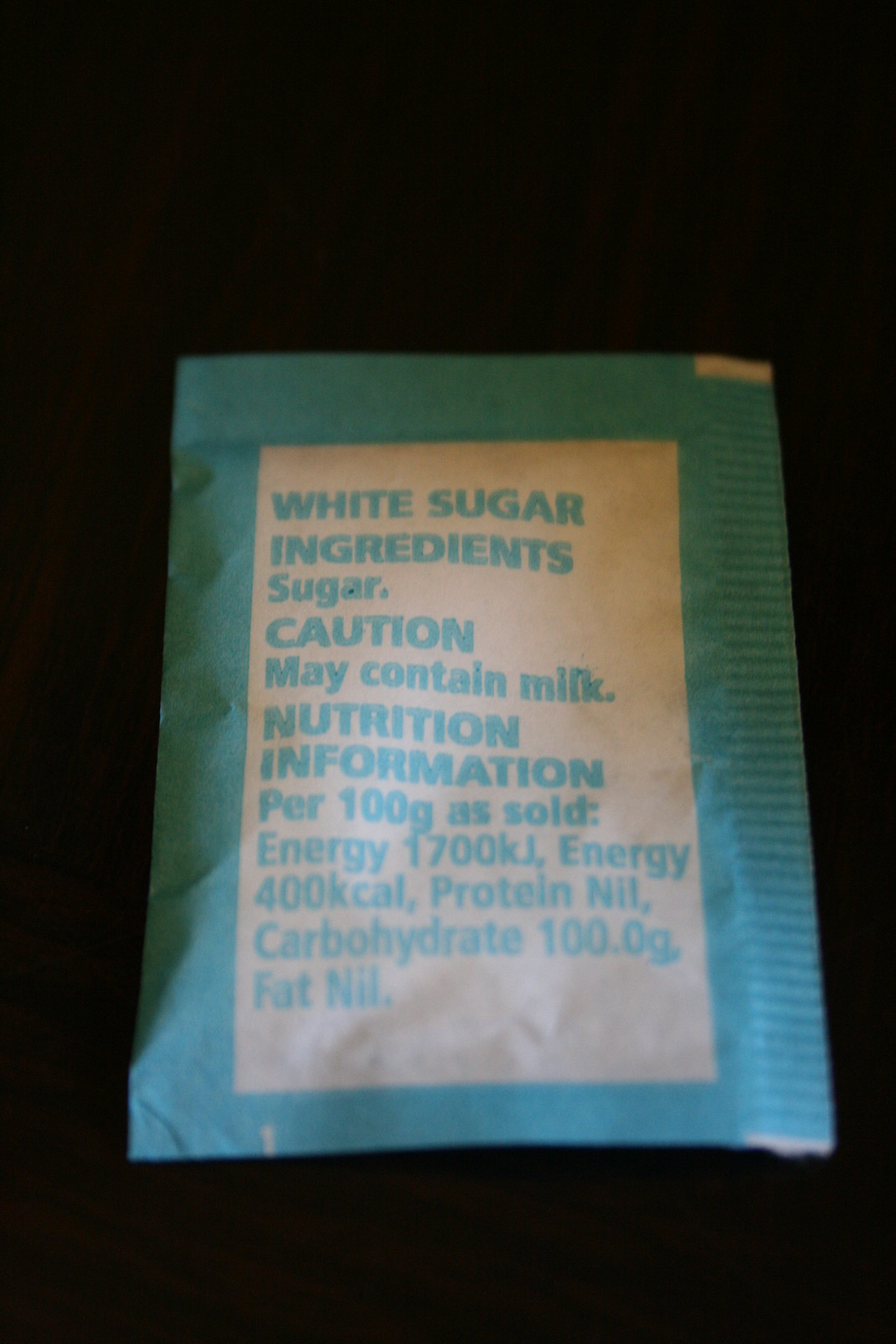This image showcases a vertically-oriented rectangular paper packet set against a black background. The packet features a central white rectangular area surrounded by a teal border, which boasts distinctive lines on the right-hand side, indicating areas designed for easy tearing. Within the white section, the text is written in teal-colored letters, prominently displaying "White Sugar." Additional details include the ingredients listed as "Sugar" with a caution that it "May contain milk." Nutritional information per 100 grams is also detailed, stating the energy content as 1,700 kJ (400 kcal), protein as nil, carbohydrates as 100 grams, and fat as nil. This packet resembles those commonly found in coffee shops, intended for individual servings of sugar.